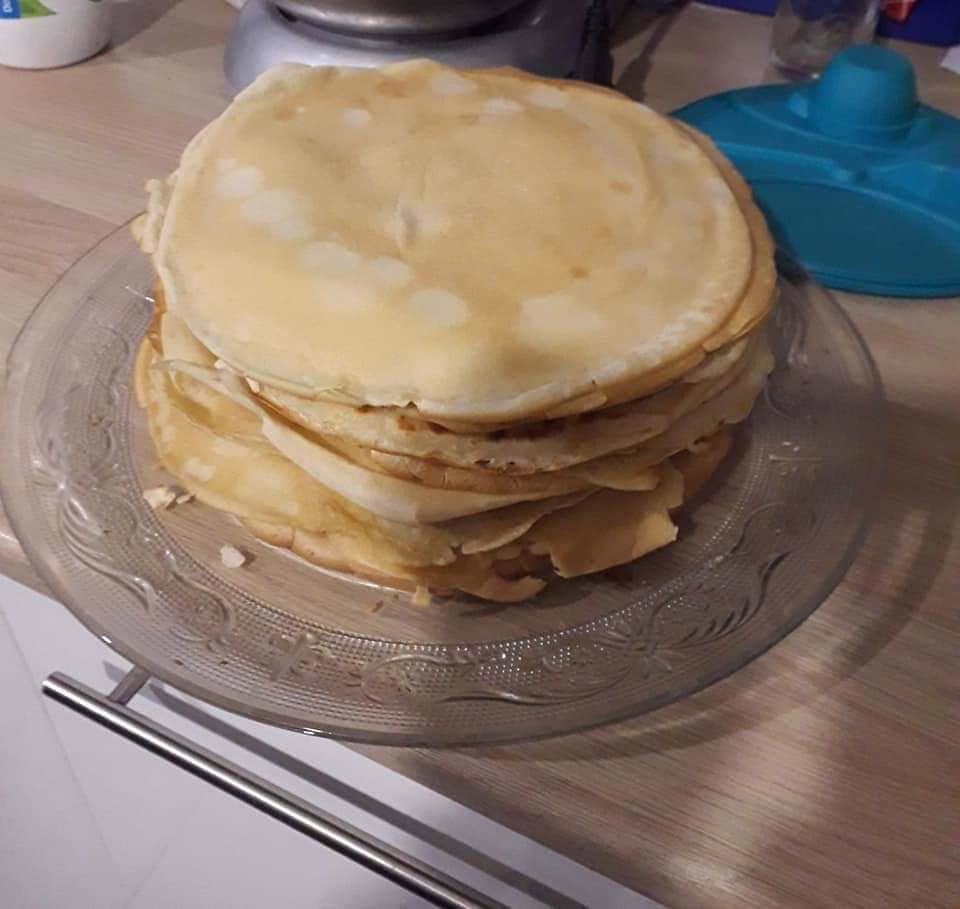In this image, we see a stack of approximately eight to ten small, very thin crepes, although they could also be interpreted as light brown pancakes. They are neatly piled on a clear, old-timey glass plate with a patterned edge. The plate is positioned on a wooden countertop, which features distinct wood patterns, and is slightly hanging off the edge by about an inch. The countertop is contrasted by a white marble-like section, possibly part of a kitchen island, with a stainless steel handle visible. The crepes themselves are a yellowy, off-white color and exhibit browning around the edges, suggesting some may be slightly overcooked. No syrup or additional toppings are present, making the stack appear plain. Behind the plate, there is a blue lid and some indiscernible metal appliances, along with a mug, indicating typical kitchen surroundings. The overall scene gives a homey, yet somewhat cluttered impression of a kitchen.